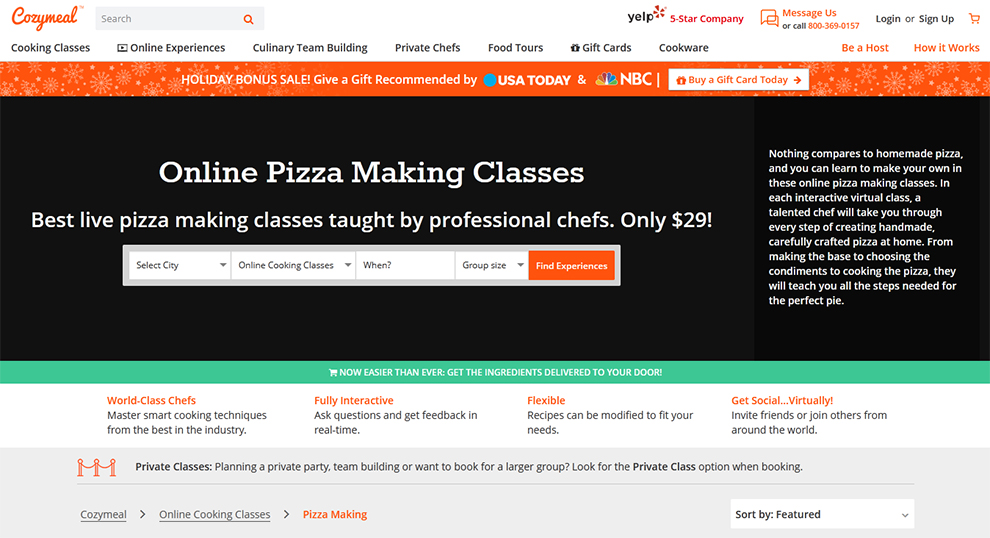The image depicts a webpage for an online application with a primary focus on promoting pizza-making classes. The screen has a predominantly black background, accentuated by vibrant touches of orange, green, and white. Central to the screen, written in white text, is the promotional message: "Online pizza making classes. Best live pizza making classes taught by professional chefs. Only $29." Beneath this message, there are functional options for users, displayed within a white rectangle with a light gray border. These options include selecting the city for the online cooking classes, specifying the date and time, choosing group size, and finding tailored experiences. Additionally, an orange patterned rectangular frame is featured at the top of the screen, emblazoned with white text that reads, "Holiday Bonus Sale. Give a gift recommended by USA Today." This frame enhances the festive appeal and suggests the classes as a thoughtful gift choice.